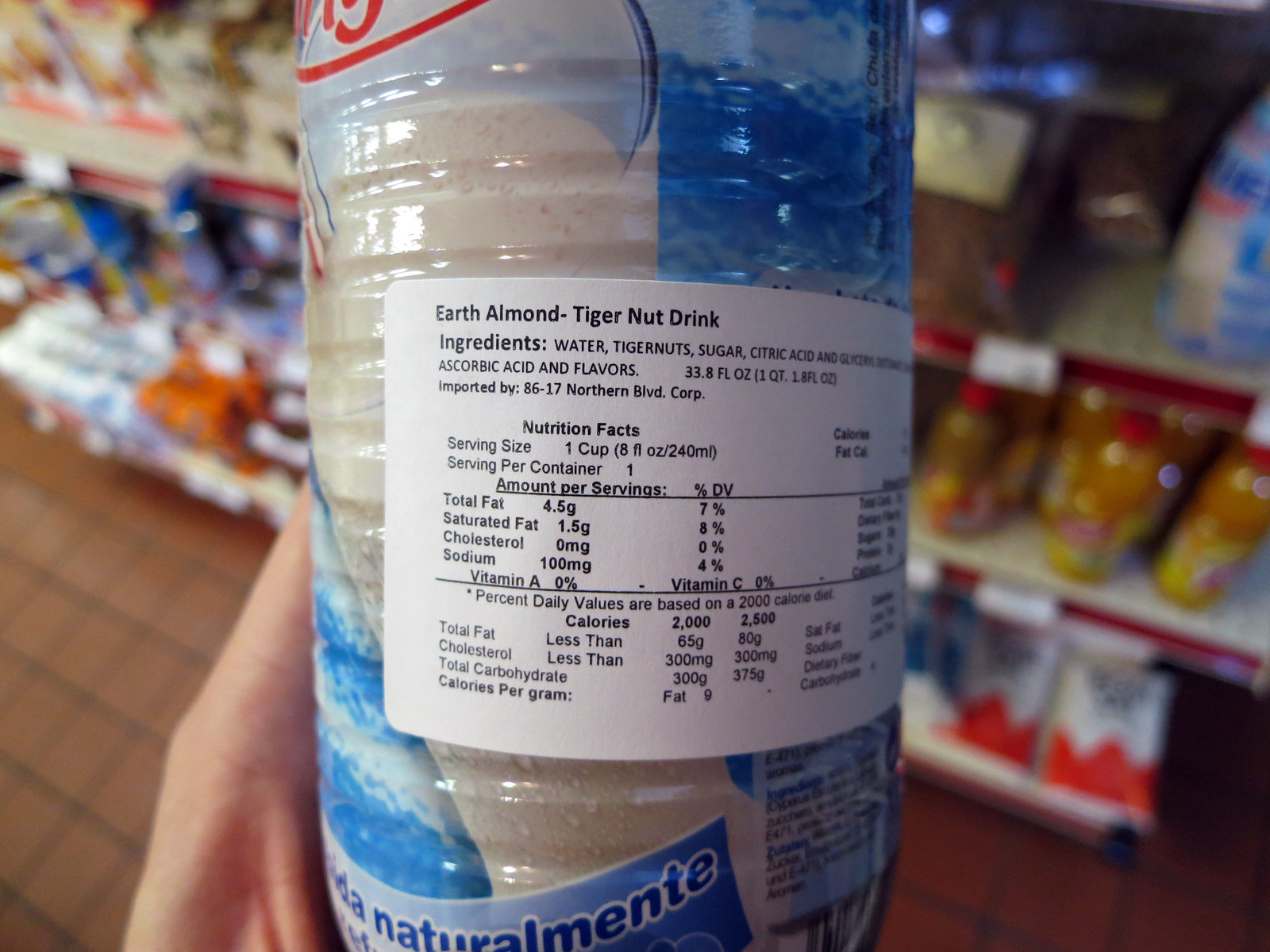The image depicts a close-up of a plastic bottle prominently labeled "Earth Almond Tiger Nut Drink," set against a blurred backdrop of a convenience store or gas station shelf stocked with various food items. The label, predominantly blue with beige accents, is the focal point of the image, offering a glimpse of the drink inside the semi-transparent bottle. Detailed on the label are the ingredients: water, tiger nuts, sugar, citric acid, ascorbic acid, and flavoring. Although partially hidden, the label also indicates the bottle's volume of 33.8 fluid ounces and includes nutritional information such as calorie content.